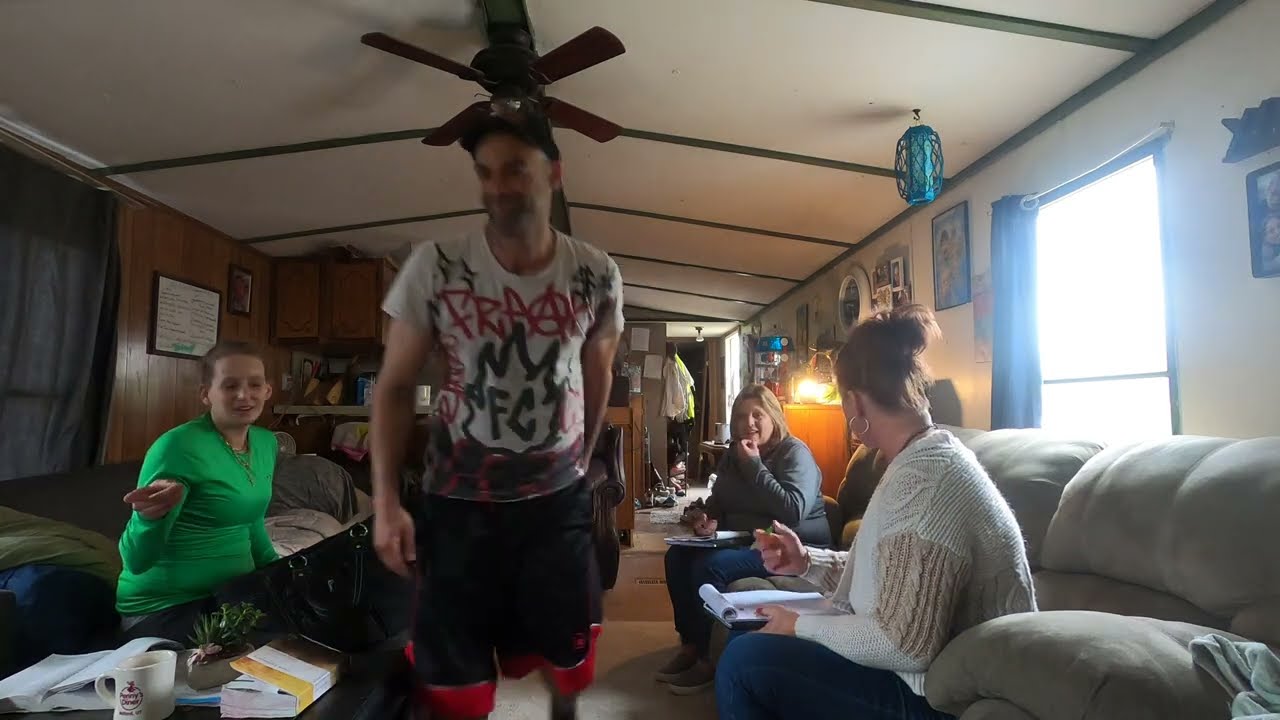The image depicts the interior of a small house, possibly a trailer, characterized by its modest and cluttered living room. At the center, a wooden ceiling fan hangs from the ceiling. Standing beneath the fan is a white male wearing a black hat, sporting some facial hair, and dressed in a white shirt with red and black spray paint-like designs, paired with black basketball shorts. He is smirking slightly while looking towards his left where a woman in a green top is seated on a couch; her eyes are closed, and she is pointing at something. 

On the opposite side of the room, two women sit on a different couch. One, seated in the foreground, has her hair tied in a ponytail and wears a white shirt. She's engaged in conversation with another woman beside her, who holds a notepad and is likely writing something down. The room features white walls adorned with a few framed pictures, enhancing its neutral and simple decor. Sunlight filters through a window behind the women's couch, illuminating the room and casting light on a table in the lower-left corner on which rests a coffee cup, some books, papers, and a small plant. In the background, a hallway is visible, cluttered with clothes hanging and other items strewn on the floor, adding to the overall busy and lived-in feel of the space.